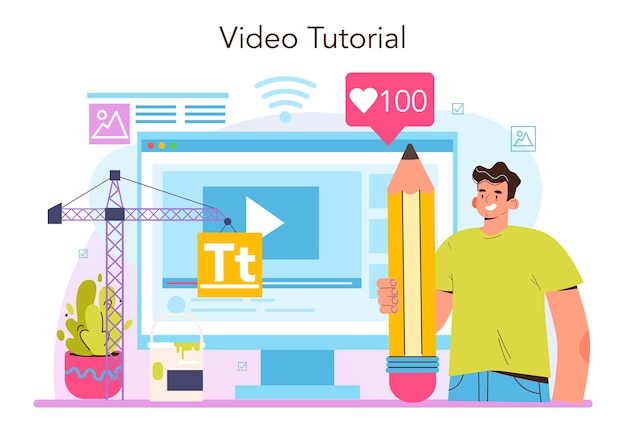This image is a computer-generated, animated illustration set against a white background, prominently captioned "Video Tutorial" in bold black letters at the top. Central to the scene is a stylized blue and white computer monitor with a large white play button on the screen. To the left of the monitor, a small purple construction crane hoists a yellow block displaying a white capital "T" and lowercase "t" underlined.

On the right side, a large cartoon man with a small head relative to his body stands outfitted in a yellow short-sleeved shirt and blue jeans. He holds an oversized yellow pencil with a pink eraser and a sharply tipped orange-and-yellow shaft, almost as tall as he is. Above the pencil's tip, a dialogue bubble contains a heart symbol followed by the number 100. Additionally, subtle details like a vase and cactus are illustrated on the left side of the image, adding to the scene's engaging composition.